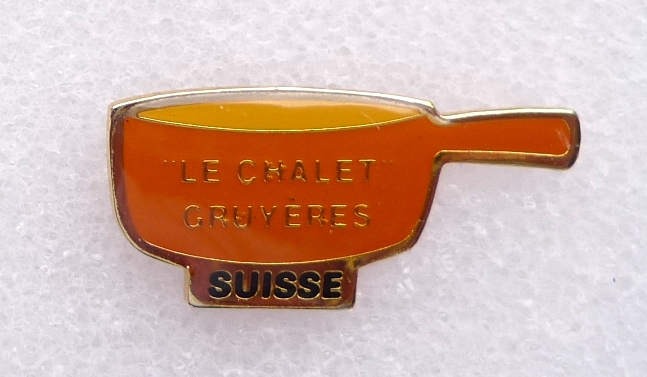The image depicts a decorative metal pin stuck into a piece of white styrofoam. This pin is shaped like a dark orange saucepan, containing what appears to be a yellow liquid. The front of the pan is decorated with gold lettering that reads "LE CHALET" in all caps. Below that, in a larger bold font, it says "GRUYÈRES." The base of the saucepan features another section with gold outlining, inscribed with black text that reads "SUISSE." This detailed and close-up photograph shows a pin that could have sentimental or commemorative value, possibly linked to a culinary context.